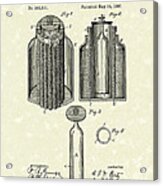This image depicts an old, extremely small blueprint, difficult to make out due to its size. It appears to be a detailed schematic for a mechanical device, possibly related to a gun barrel or bullet chamber. The top portion showcases the front and back views of a cylindrical structure, reminiscent of a sarcophagus with one side facing forward and the other backward, accompanied by illegible notes. The bottom section of the blueprint features a cylindrical figure narrowing at the top, potentially the inside of a barrel, with a small gray circle adjacent to it and another pointed shape below. Various measurements and diagrams are scattered across the blueprint, though they are too small to decipher. Overall, the blueprint combines illustrations and notes, presenting the initial design specs of the mechanical parts involved.